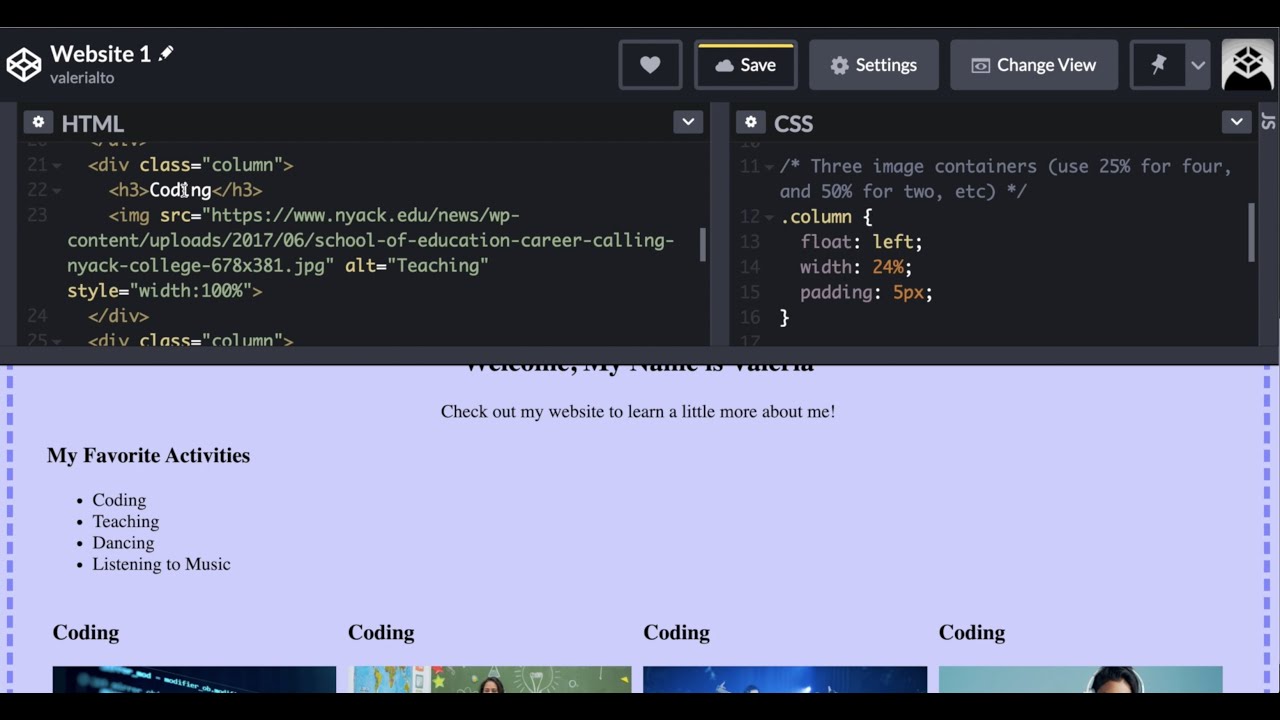A detailed screenshot from a coding interface showcases a variety of elements. The top half of the page features a sleek black background with white text. Positioned in the upper left corner is a 3D rendering of a square box, beside which the labels "Website 1" and "Valeria Alto" are displayed. Moving rightward to the center of the page, there is an icon of a white heart inside a square, followed by a rectangular button labeled "Save" accompanied by a cloud icon. Adjacent to this is a gray rectangular button housing a small gray gearbox icon and the text "Settings." Next, there is another rectangular button labeled "Change View," succeeded by a thumbtack icon with a drop-down menu.

Below this toolbar, the content section begins with HTML coding elements, accompanied by drop-down menus. To the right, there is a small gearbox icon followed by the label "CSS" and another drop-down menu. Further down, the page displays image containers with specified usage percentages: 25% for four images and 50% for two images, succeeded by additional coding.

The bottom portion of the screenshot features a light lavender background with black text stating, "Welcome, my name is Valeria. Check out my website to learn a little more about me." To the left, a list of Valeria’s favorite activities is presented: coding, teaching, dancing, and listening to music.